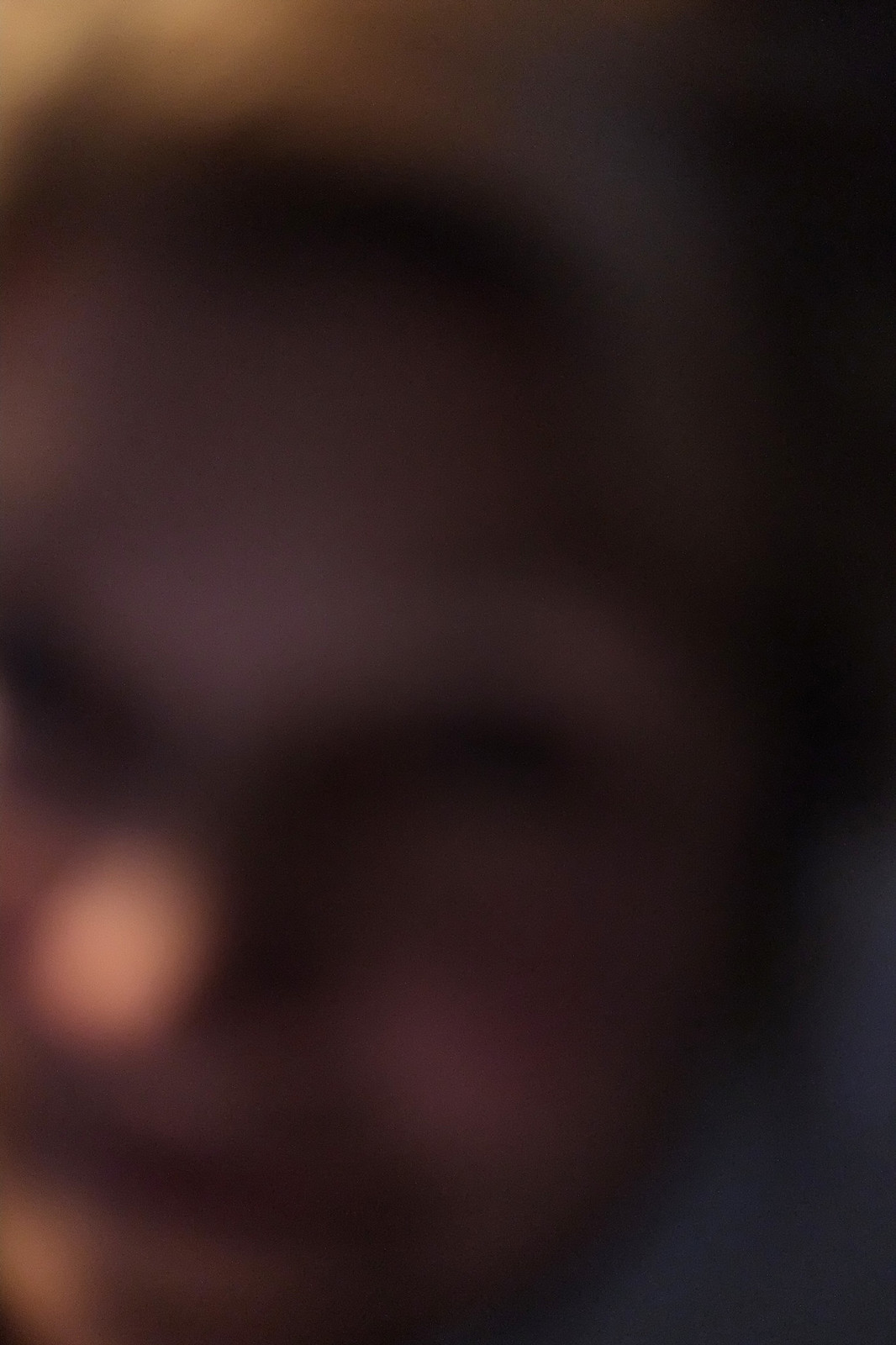In this image, we see a predominantly dark, blurry photograph that is out of focus. The right and lower corner are filled with a solid black background, while the upper left corner and portions of the lower left side exhibit subtle hints of illumination attempting to break through the haze. In the center-left and bottom-left regions, as well as the left side towards the middle, there are lighter gray areas that suggest an effort of light struggling to emerge. The right side remains a deep, uninterrupted black. The image features three distinct areas of light on the left side: two in the bottom left corner and one towards the top left. Additionally, a broader, lighter gray area appears in the center-left portion of the image, hinting at light trying to penetrate the pervasive darkness and blur.